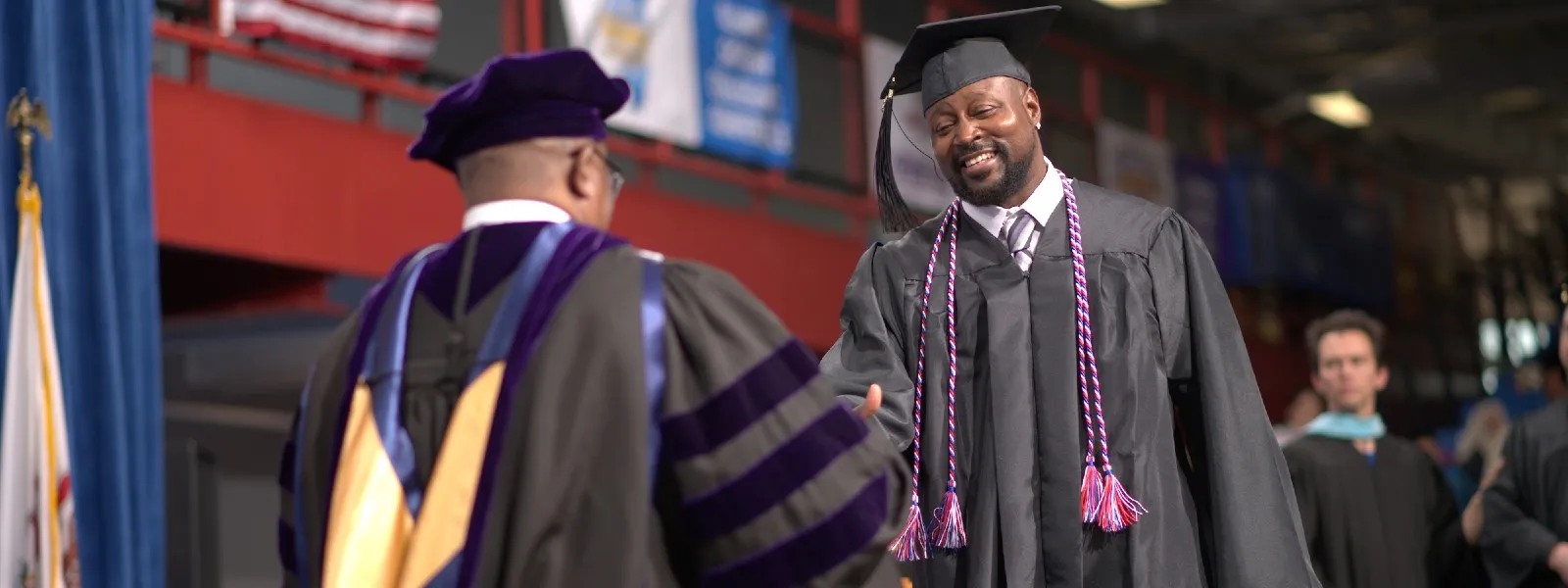This detailed color photograph captures a moment at a graduation ceremony. On stage, two African American men are engaging in a handshake. The man on the left, likely a professor, is shown from behind, wearing a black robe adorned with three distinctive purple stripes on his right arm and a purple hat. In contrast, the man on the right, a graduate, is oriented towards the camera. He sports a black graduation cap with a tassel hanging to the right, a black robe, and distinctive dual-colored braided ropes—purple and red—draped around his neck.

In the background to the right, a Caucasian man with black hair is visible. He also wears a black graduation robe, complemented by a blue scarf around his neck but lacks a hat. The setting is further detailed with a blue curtain and a red balcony adorned with banners in the backdrop. Additionally, there is an American flag partially visible and a small white flag in the left-hand corner. A crowd of onlookers is hinted at on the right side of the image, adding to the celebratory atmosphere of the graduation ceremony.